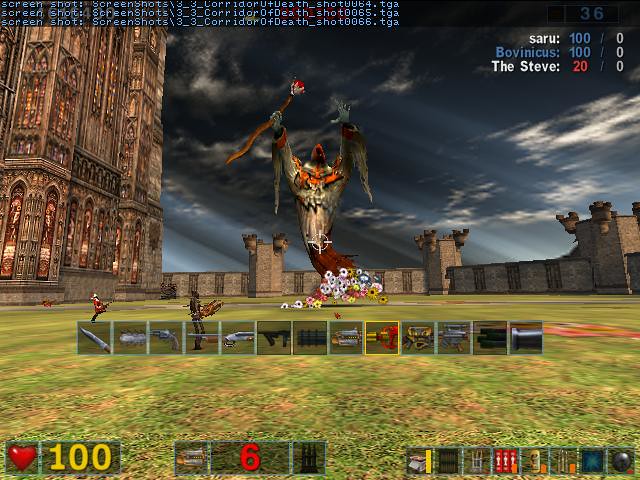This detailed screenshot, captured from the video game "Corridor of Death," showcases an intense in-game scene displayed on a computer monitor. The image prominently features a towering, menacing monster standing next to a grand structure reminiscent of the Notre Dame cathedral. This imposing castle is set within a vast lawn, surrounded by a formidable fortress in the background.

The scoreboard at the top lists three players: Saru and Bonavicus, both with 100 points, and TheSteve, who has 20 points. In the scene, a colossal monster, wielding a scepter, appears to have just defeated another creature, adding to the dramatic atmosphere. The setting is vibrant, featuring a rich palette of bright blues, blacks, greens, yellows, and browns. Smaller figures, possibly armed, are scattered across the lawn, adding further intrigue to the battle unfolding in this immersive gaming landscape.